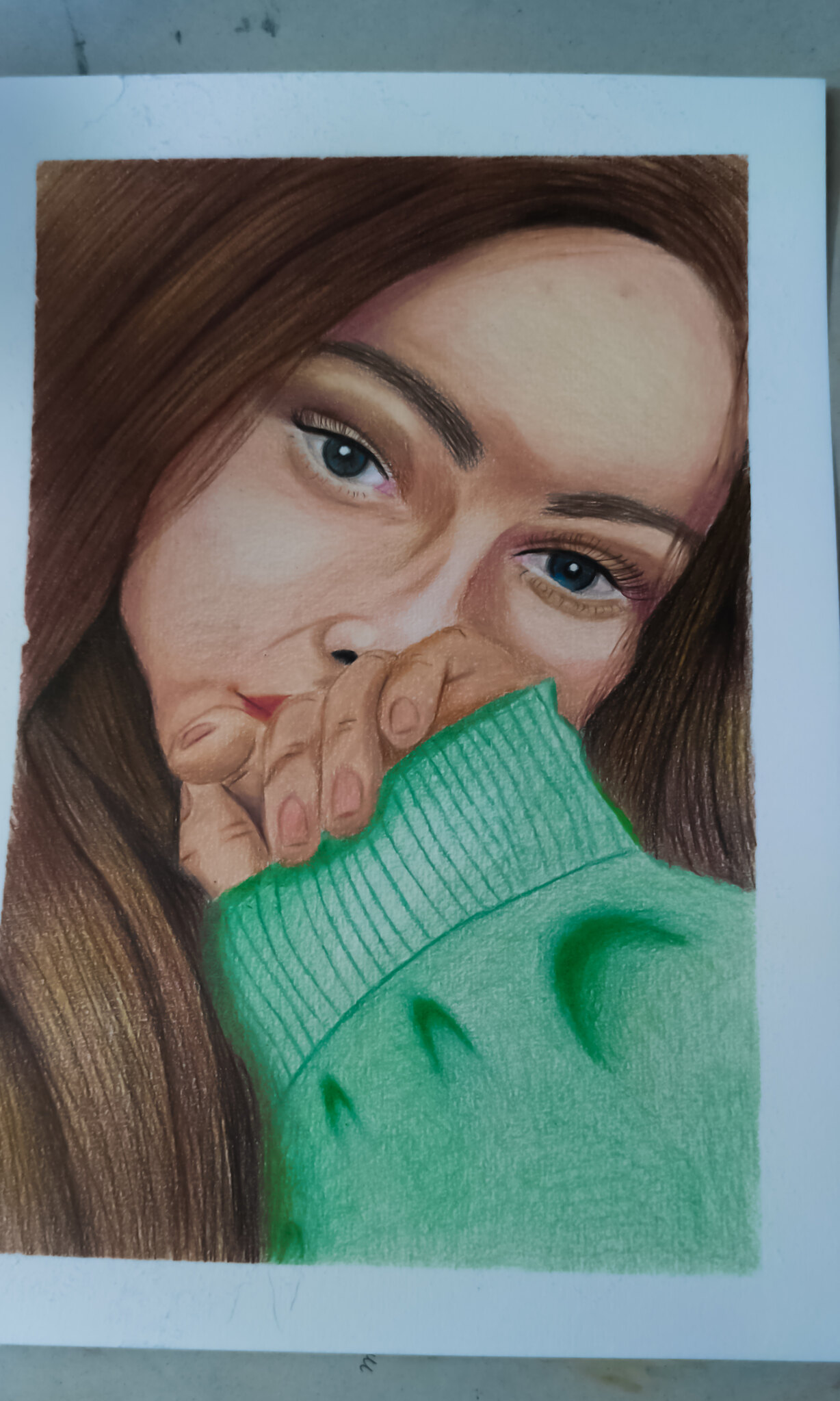This illustration depicts a woman rendered in what appears to be colored pencil. She gazes subtly towards the viewer with captivating dark blue eyes, her head tilted slightly to the right. Long, flowing brown hair frames her face. Her left hand is raised partially in front of her face, covered by the sleeve of a green sweater, which is pulled up slightly, revealing fingers and detailed wrinkles in the fabric. The entire illustration is encased in a white border, and the bottom portion reveals the edge of a white table beneath.